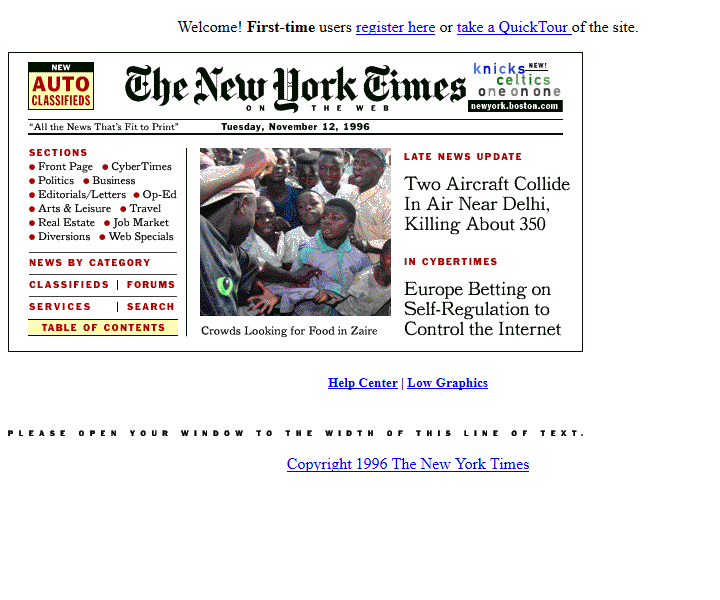The image is a screenshot of a website displaying an emulation of a New York Times newspaper. At the top right corner of the page, there is a user prompt that reads, "Welcome, first time users, register here or take a quick tour of the site," with the phrases "register here" and "take a quick tour" both appearing as blue, underlined hyperlinks. 

Beneath this prompt, a mock-up of a traditional New York Times newspaper is featured prominently. The newspaper's iconic black-lettered masthead, "New York Times," is displayed at the top in an old-fashioned font. Flanking the mock-up on both left and right sides are advertisements—one for auto classifieds and the other for a segment titled "Nic's Celtics One-on-One."

Central to the mock-up is a photograph capturing a group of people huddled together, presumably in a conflict situation. The caption beneath the image reads, "Crowds looking for food in Zaire." 

On the left side of the page, a navigation menu offers various sections of the paper including "News by Category," "Classified," "Forum," "Services," "Search," and "Table of Contents."

To the right of the mock-up, two prominent news stories are featured:
1. "Two aircraft collide in air near Delhi, killing about 350."
2. "You're betting on self-regulation to control the Internet."

Additionally, there are links to "Help Center" and "Low Graphics" for further assistance.

At the very bottom of the page, the text reads, "Copyright 1996, The New York Times," indicating the content's year of copyright.